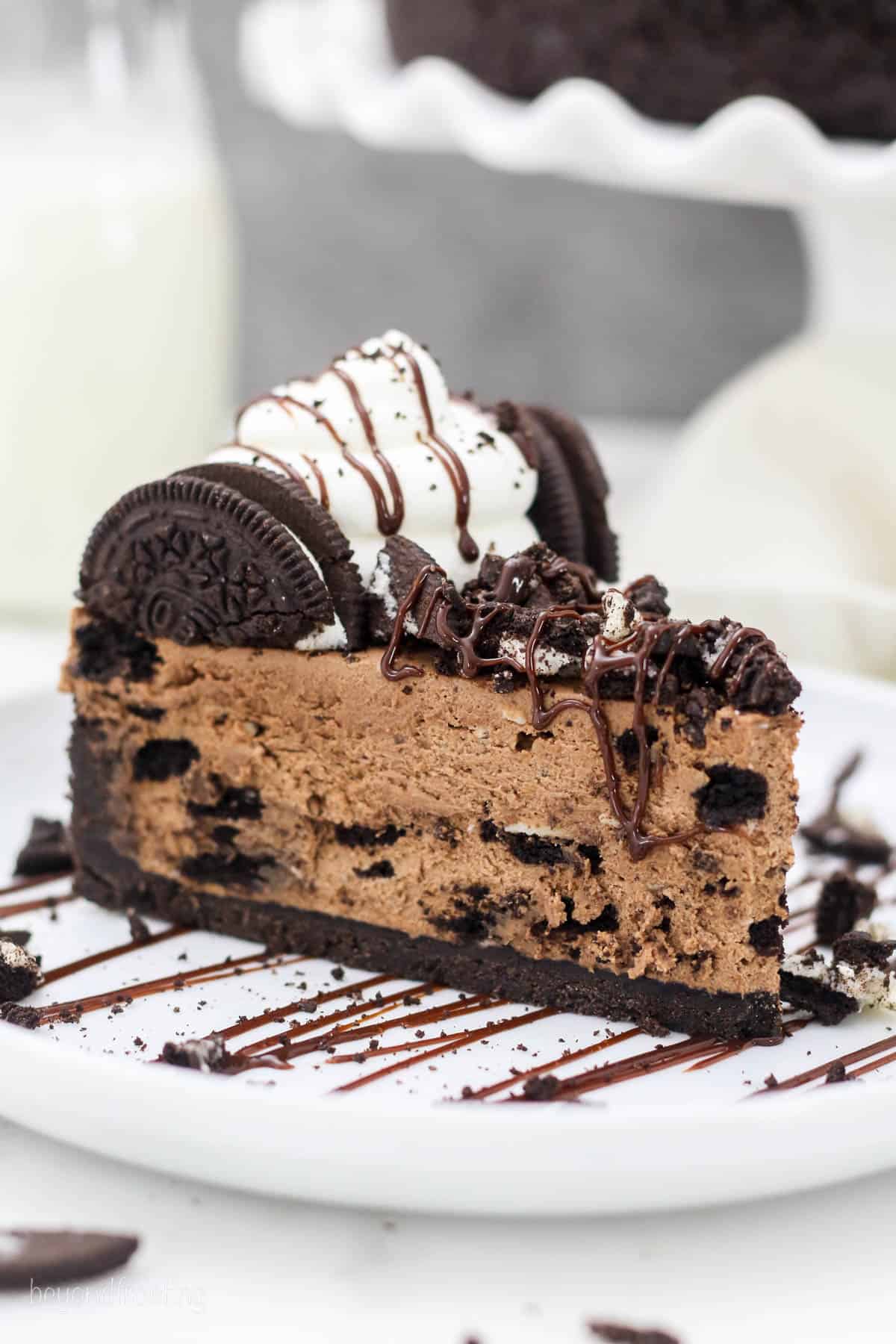This vertical rectangular close-up image showcases two decadent pieces of chocolate dessert on a white round tray. The foreground focuses on a slice of chocolate cheesecake with a black cookie base, its light chocolate filling flecked with bits of Oreo, and adorned with a dollop of whipped cream covered in chocolate sauce and topped with Oreos. The plate beneath features a zigzag pattern of chocolate syrup and scattered chocolate crumbs, enhancing the visual appeal. Slightly blurred in the background, partially obscured by the cheesecake, is a likely chocolate éclair topped with white frosting and drizzled chocolate. The background blur reveals hints of more white china, a cake stand with a dark cake, a glass bottle of milk, and additional chocolate pieces on the table, drawing attention to the rich, inviting desserts prominently displayed.